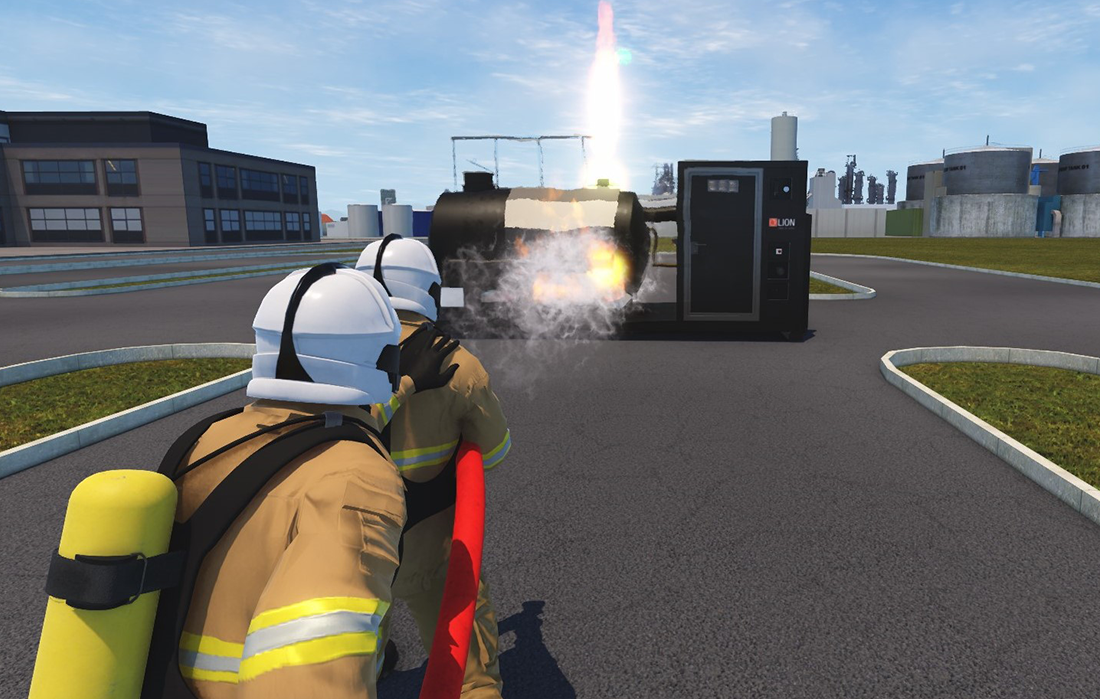In this detailed video game simulation image, two firefighters clad in brown uniforms with high-visibility reflective stripes and white helmets adorned with black stripes are depicted in the foreground. They stand on a paved road bordered by white trim and interspersed with patches of grass. The firefighter in front grips a red hose under his right arm, directing a spray toward a blazing, black object suspected to be an exploded gasoline or propane tank in the middle of the scene. The second firefighter, equipped with a yellow oxygen tank, steadies his left hand on the first firefighter's right shoulder, offering support. Surrounding them is a multi-story office building to the left, an assortment of oil drums and utility barrels to the right, and an industrial area in the distance, all beneath a clear blue sky with some clouds.